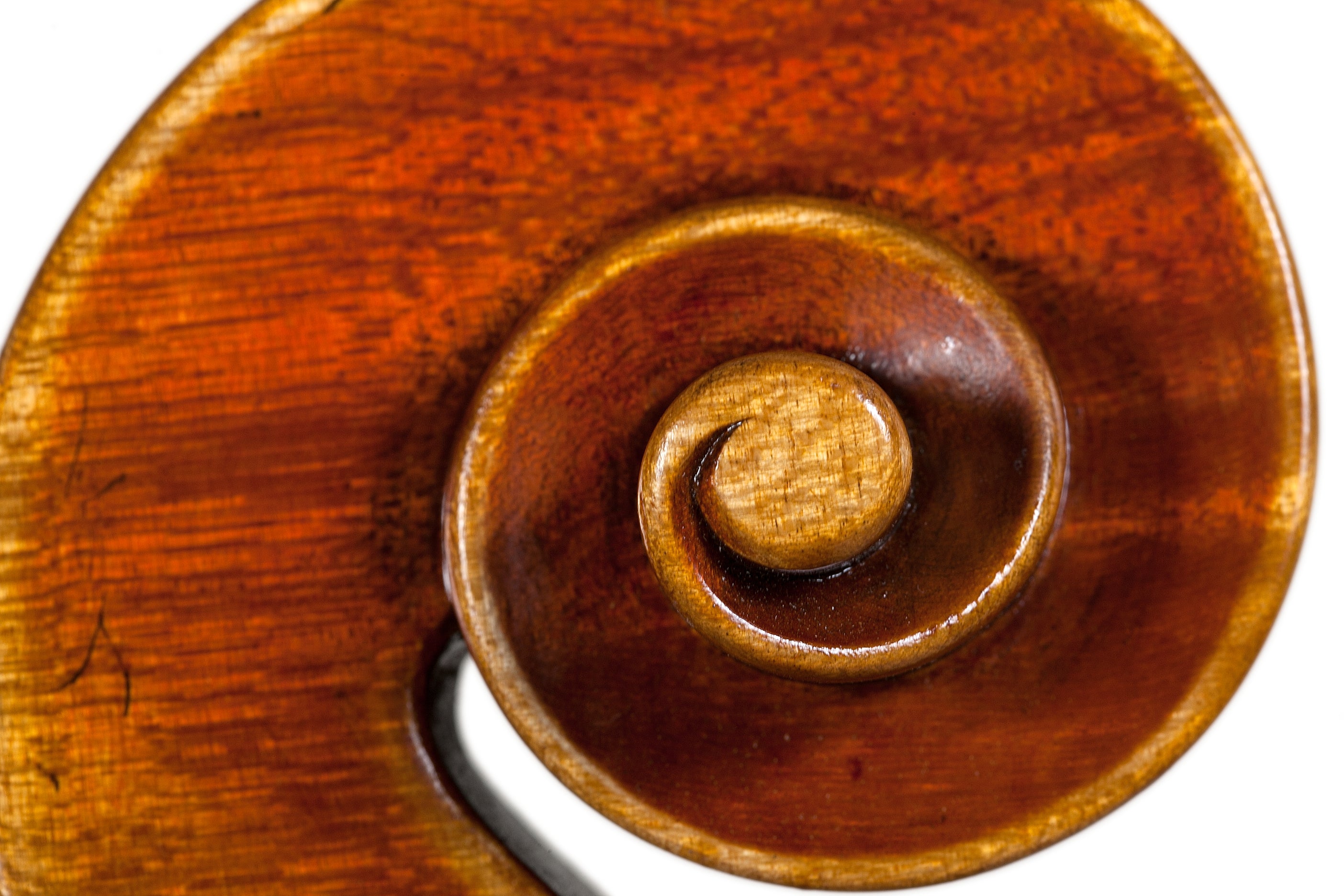In this photograph, we observe a close-up of a fingerboard head from a string instrument, likely a cello or violin, emphasizing the detailed craftsmanship of the wood. The head features a decorative spiral curl that begins in the bottom left, ascends in a clockwise motion, and curves inward to form a swirl reminiscent of a comma or apostrophe. The outer part of the wood showcases a lighter yellowish-brown hue, while the inner areas of the swirl dip into a deeper, darker brown, suggestive of mahogany. The piece appears worn and slightly dusty, with visible dust particles and black scratches or marks near the bottom left corner. This close-up, set against a stark white background, isolates the wooden head, casting a subtle shadow and providing no additional context for the object's size or surroundings. The entire piece, stained and lacquered, captures the delicate artistry in what might initially seem a purely decorative element.